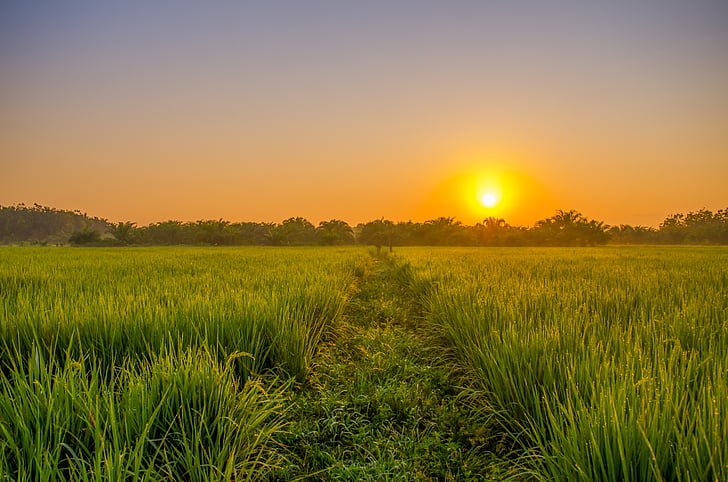The photograph captures a serene, expansive landscape of a large, green grassy field at golden hour, just as the Sun is positioned at the horizon, casting its final glowing rays. The sky above transitions from a deep bluish purple at the top to a medium orange nearer the horizon, creating a breathtaking gradient that highlights the beauty of the scene. In the foreground, tall, vibrant green grass sways with life, standing at about six inches to a foot in height. Cutting through this tall grass is a distinct, narrow pathway, either mowed shorter or trampled down, leading the eye towards a diverse line of trees in the distance, with a few low hills framing the view. The Sun, a bright yellow orb, is captured in the throes of setting, its light casting a warm, golden hue across the field. The distant trees, likely a mix of palms and others, add a subtle boundary to the expansive meadow, emphasizing the natural beauty of this moment of transition from day to night.